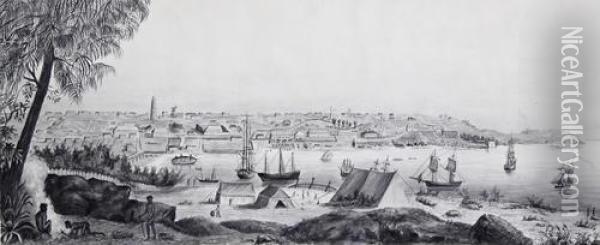The image depicts a black-and-white line drawing, likely a piece of fine art created with pencil or charcoal shading. It illustrates a broad, panoramic view of a large harbor, evocative of an old-world scene reminiscent of perhaps Boston Harbor. Distinct elements include numerous sailing ships, some with sails raised and some without, floating on the water near a pier. A town stretches from the water's edge to the horizon, with low buildings punctuated by a few tall spires. The waterfront is adorned with rows of trees. 

In the foreground, an indigenous settlement is visible, characterized by large tents and people tending to campfires. Among these figures, one person is seated under a tall tree on the left, with another figure seemingly crawling towards them, and a third figure standing behind. The presence of large rocks adds to the landscape's rustic elements. The scene also reveals a background featuring indistinct, possibly blurry and fuzzy structures and a low mountain peninsula to the right. The right-hand side of the artwork bears a watermark that reads "NiceArtGallery.com".